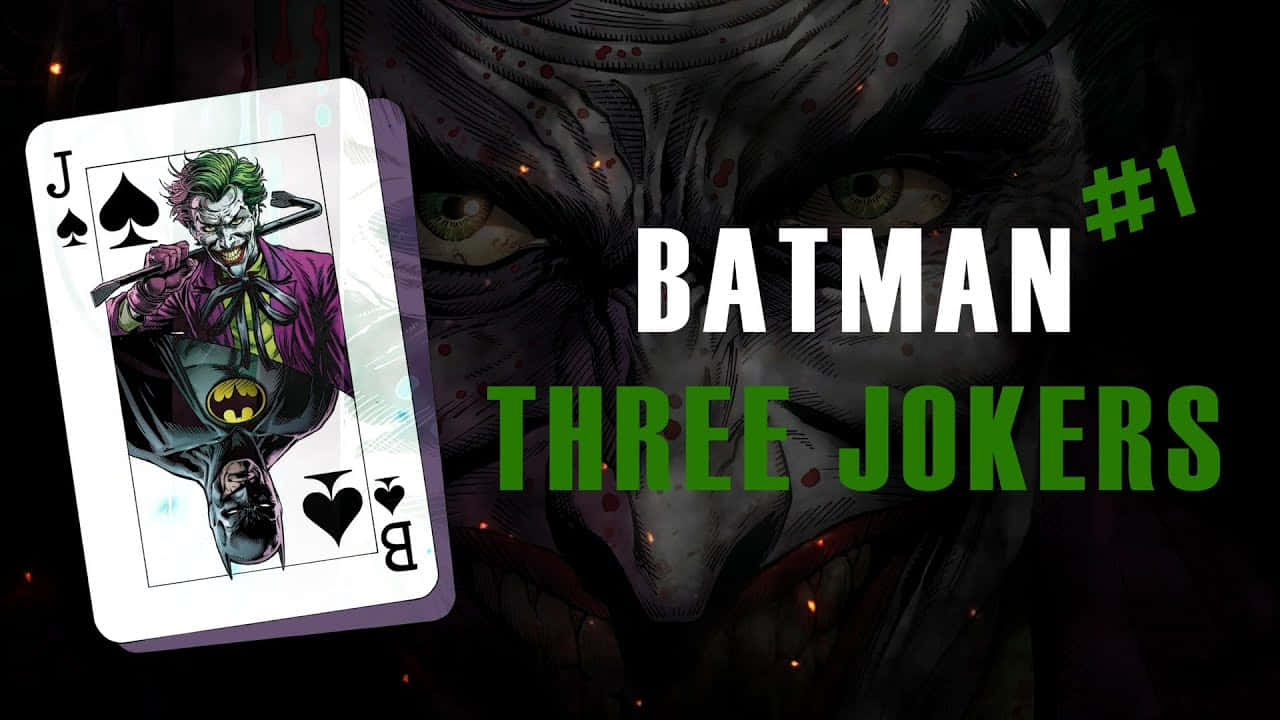This image is an advertisement, likely for a comic book titled "Batman: Three Jokers Number One." The background is very dark and showcases a detailed, close-up image of the Joker's face, with intense green eyes, red lips, and prominent wrinkles, giving him an eerie, menacing look. Overlaying this backdrop, "Batman" is written in white letters, and below it, in green lettering, are "#1 Three Jokers."

On the left-hand side of the image, there is a prominent playing card from a deck of spades, featuring the Joker and Batman. The top half of the card shows the Joker, adorned in his signature purple long-sleeved jacket and bright green hair, holding a crowbar over his shoulder. The bottom half, inverted, depicts Batman in his traditional black suit with the yellow emblem on his chest. The card designates the Joker's side with a "J" and Batman's with a "B". The flip side of this card, visible behind it, is purple.

The overall composition gives a gloomy and intense feel, emphasizing the dark and twisted relationship between Batman and the Joker.